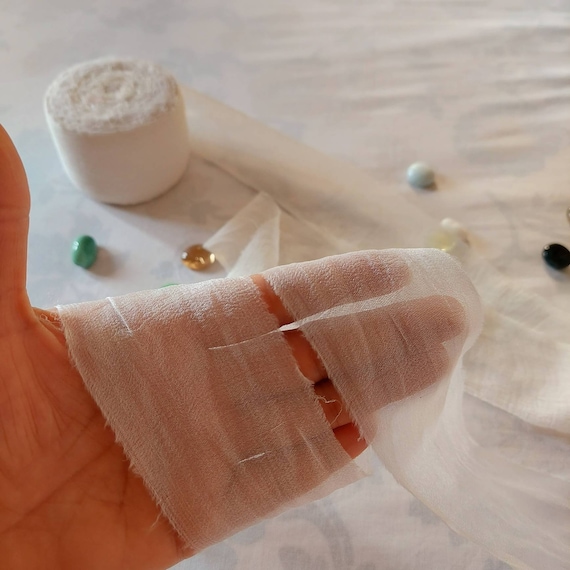The photo depicts a person's left hand, open with the palm facing the camera, wrapped in medical gauze around four fingers, leaving the thumb unwrapped and pointing upward. The gauze appears to be part of an unraveled roll in the background at the top left. The scene is set against a white background. Scattered near the hand are several multicolored small objects, each resembling gems or possibly candy. These include a turquoise gem resembling a jelly bean, a gold gem beside it, a white gem ball with a yellowish-clear gem below it, and a black gem ball further to the right. The gauze wrapping the hand shows a small break between the fingers, indicating a delicate and meticulous wrap.